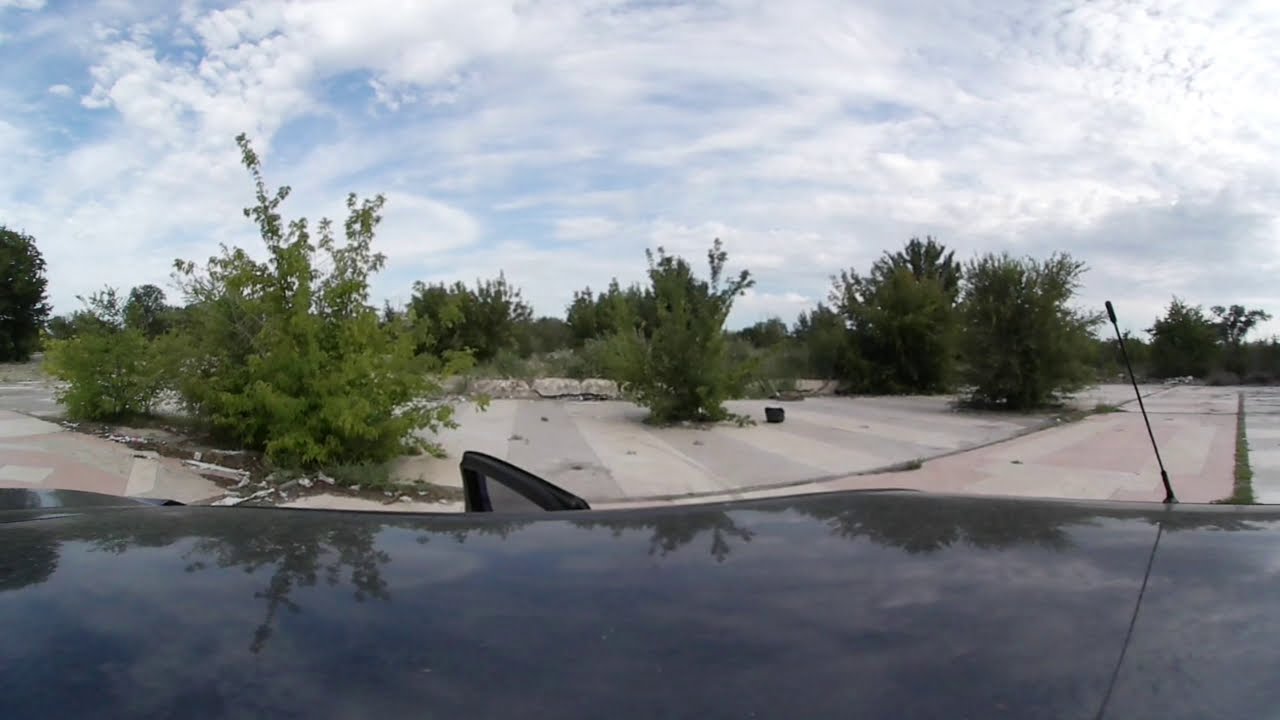The photograph, taken with a fisheye lens during the daytime, captures an outdoor scene from the roof of a black SUV, identifiable by its antenna and the driver's side door slightly ajar on the left. The lower half of the image reveals the roof of the vehicle, while the upper half showcases a desolate, overgrown parking lot. The ground, composed of cracked concrete, has been overtaken by nature, with large green trees and dense bushes sprouting up through the fissures. The background stretches out into an expanse of more trees and vegetation, suggesting a once-maintained area now abandoned. Scattered debris is visible on the right, further emphasizing the neglect. Above, a blue sky is filled with numerous white clouds, adding a contrasting serenity to the scene.